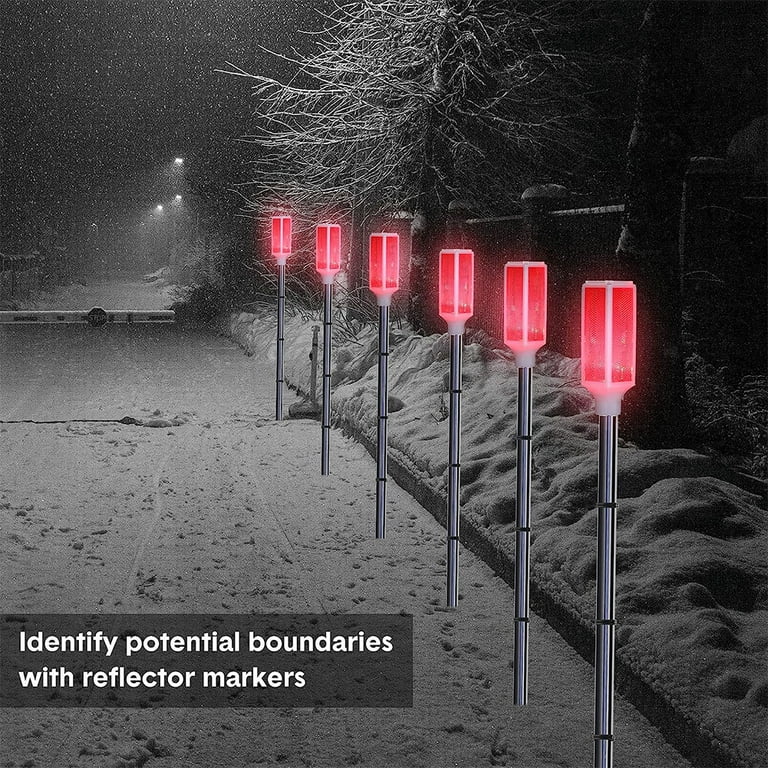This computer-generated, black-and-white image depicts a snowy winter night on a street, primarily aimed at showcasing the use of reflector markers. On the right-hand side, there are six metal poles with red rectangular lights perched on top, arranged parallel to the snow-covered sidewalk, which features minor snowy hills along its edge. There is a leafless tree on the sidewalk, and further into the background, some street lamps are visible. On the bottom left corner, the image includes a semi-transparent black border with white text that reads, "Identify potential boundaries with reflector markers." These reflector markers are clearly emphasized to highlight their role in delineating the sidewalk's edge for drivers amidst the heavy snowfall.